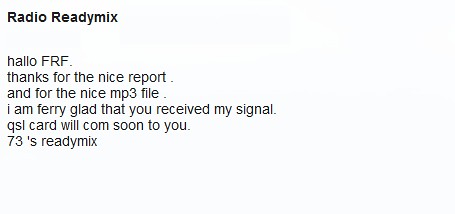In the image, there is black text on a white, slightly off-white background. The primary heading at the top is bold and larger, stating "Radio Ready Mix." Below this, there are six lines of regular text, slightly indented to the left. The first line reads "HALLOFRF" in all capital letters. The following lines respectively say: "Thanks for the nice report.", "And for the nice MP3 file.", "I am very glad that you received my signal.", "QSL card will come soon to you.", and finally, "73's Ready Mix." The overall appearance resembles a business card or postcard from a radio station, emphasizing the text without any additional imagery or borders.